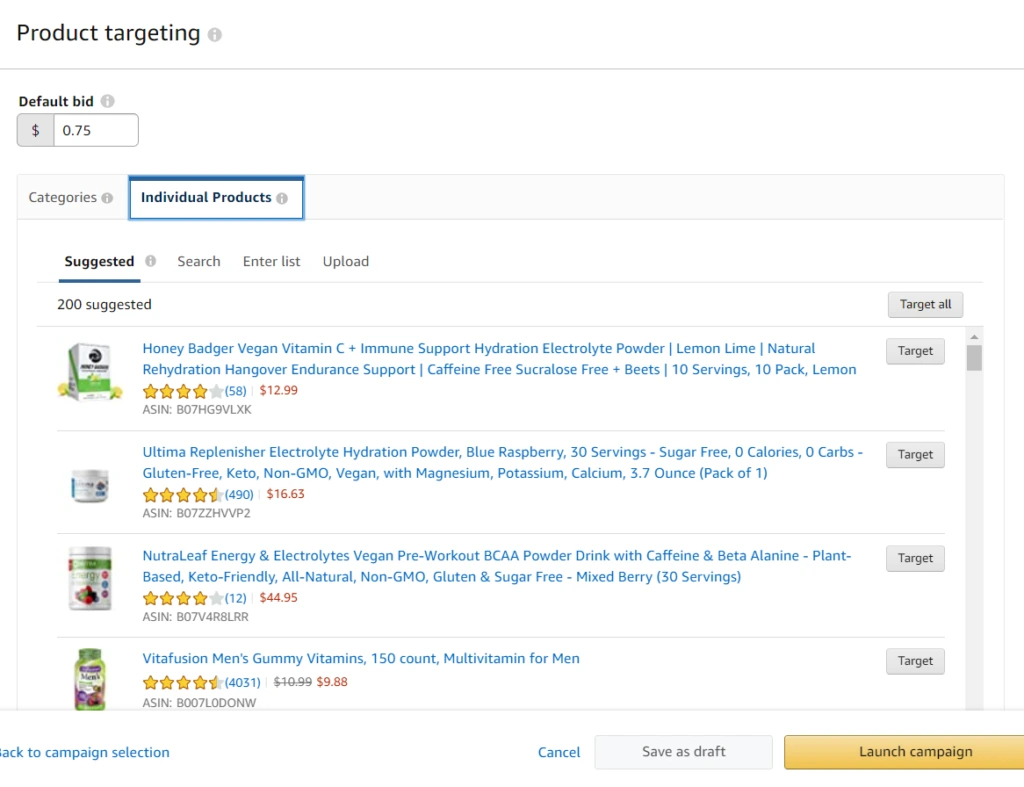The image depicts a detailed view of a website interface designed for product targeting. In the top left corner, there is a heading titled "Product Targeting" set against a white background, accompanied by an information icon to the right for additional details. Beneath this heading, a fine grey line spans the width of the screen, serving as a separator.

Directly below the line is a field for entering a default bid, which is currently set at $0.75. This section is followed by a light grey panel featuring two selectable tabs labeled "Categories" and "Individual Products." The "Individual Products" tab is currently selected.

Underneath the tabs, there are several subheadings: "Suggested," "Search," "Enter List," and "Upload." The "Suggested" subheading is highlighted, revealing a list of 200 suggested items. These items are displayed along the left side of the screen, each accompanied by a thumbnail image, product title, star rating, price, and a unique SIN (Stock Identification Number) reference.

To the right of each product listing, there is a target button available for users to click if they wish to target that specific product. At the bottom right corner of the screen, a prominent yellow button provides an option to launch a campaign with the selected targeted products. Alternatively, users can choose to cancel or save their progress as a draft.